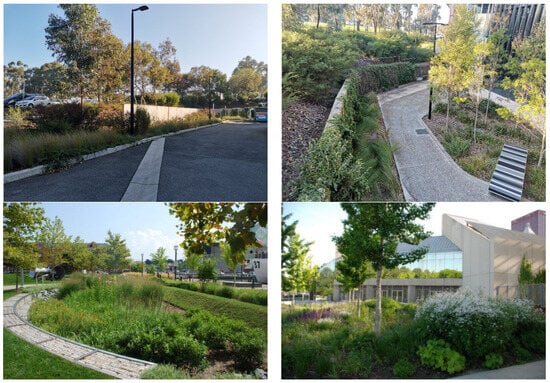This image is a composite of four separate shots, each occupying a quarter of the total frame, and appears to be taken from security camera feeds showing various outdoor scenes with pathways, greenery, and structural elements. The top left section features a streetlight along a roadway with a wall and parked cars visible behind a line of trees in the background. The top right section provides an overhead view of a pentagon-shaped courtyard with a concrete hexagonal walkway surrounded by a wall, trees, and shrubs both inside and outside the enclosed area, and distant buildings visible. The bottom left section depicts a small neighborhood park with a round walkway encircling bushes and green shrubs, with houses and additional greenery in the background. The bottom right section prominently shows a building with angular sides and reflective glass siding; in front of this structure, there is a thick bush and several small trees. Notably, there are no people visible in any part of the image.